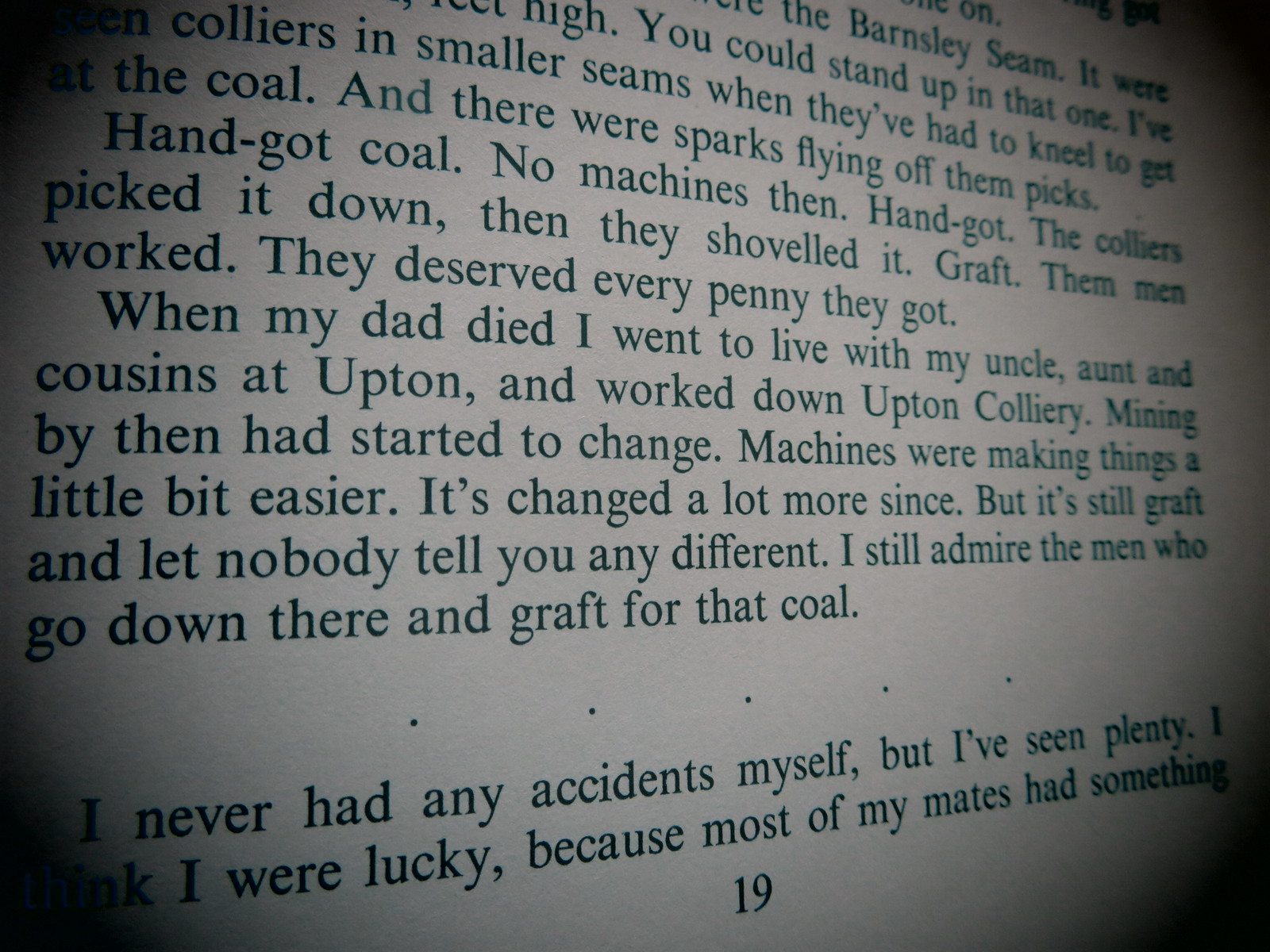The image depicts a slightly turned page from a book, with the right side appearing farther away than the left. The top of the page is cut off by the image's frame, making it impossible to see the complete text. The page, marked as number 19 at the bottom, contains several sections of black printed text. The first block of text consists of several lines, followed by an indentation and three more lines of text. Another indentation leads to six more lines of print. Midway down the page, a space with five horizontally spaced dots further divides the text. Below this dotted line, there are two additional lines of text. The legible portion reads: "When my dad died, I went to live with my uncle, aunt, and cousins at Upton, and worked down Upton Colliery. Mining by then had started to change. Machines were making things a little bit easier. It's changed a lot more since, but it's still graft, and nobody tell you any different. I still admire the men who go down there and graft for that coal." The image cuts off some text at the top and bottom, and the visible text is somewhat hard to read due to the angled capture of the page.